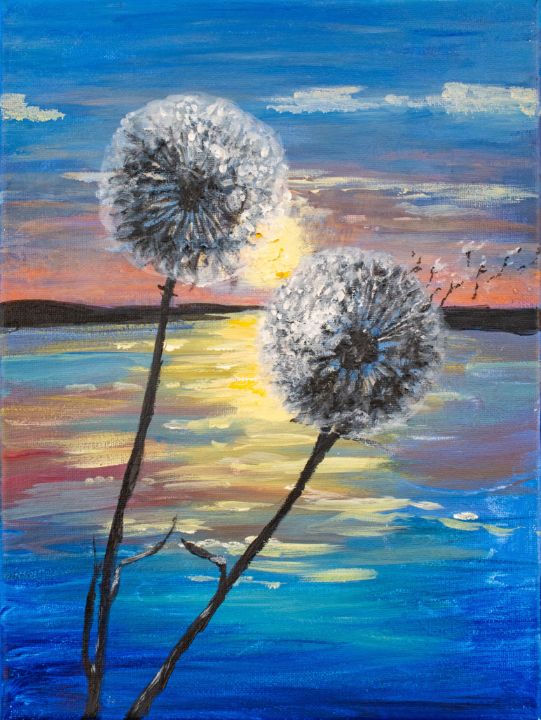This oil painting vividly captures the serene beauty of a sunset. The sky, transitioning from blue at the top to vibrant hues of orange, yellow, and light pink, is adorned with thin white clouds drifting across. The sun, a radiant yellow orb positioned near the center of the horizon, illuminates the scene with its golden glow. Below the horizon, a peaceful lake or river mirrors the stunning sky, with shimmering ripples reflecting the sun's light in vibrant blue and yellow tones. The foreground features two delicate dandelions with brownish-black stems, their white, spherical seeds gently drifting away in the breeze. The painting evokes a sense of calm and fleeting beauty, capturing the timeless moment of sunset.